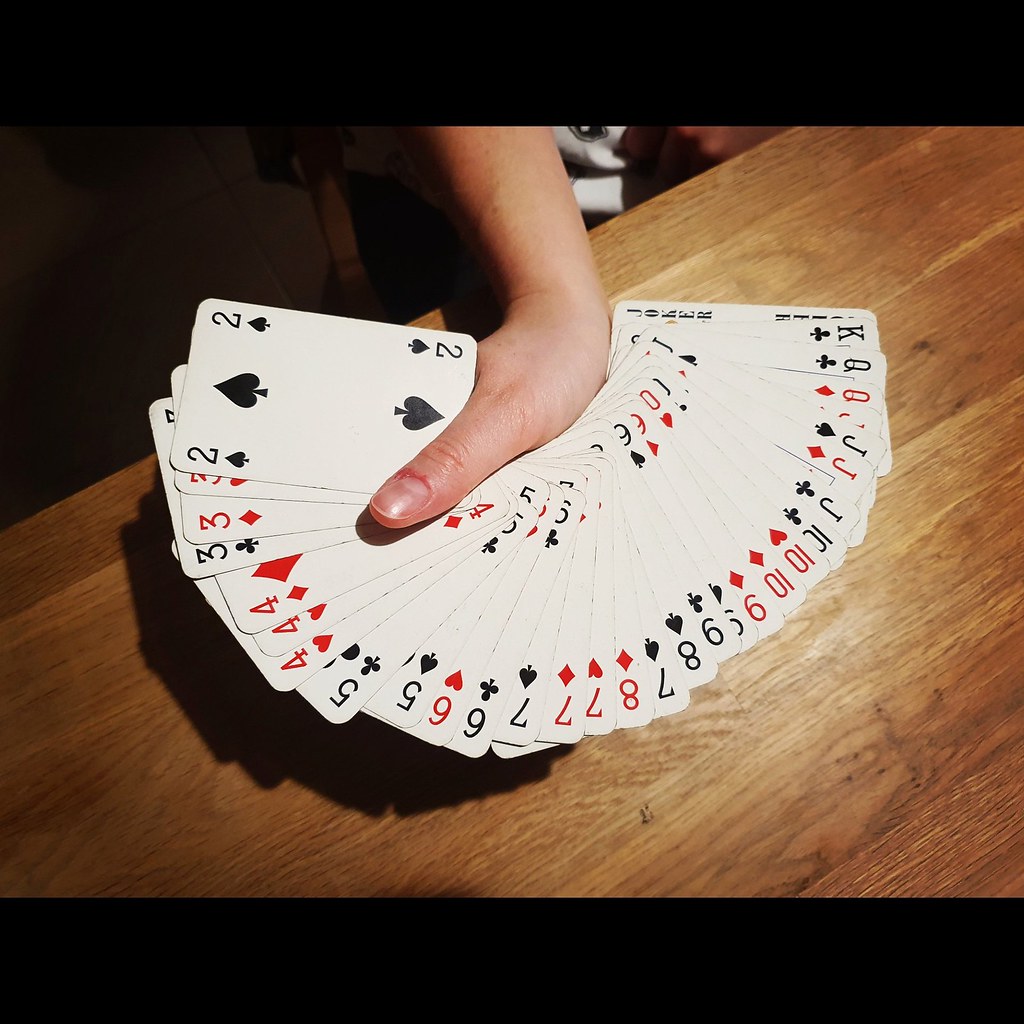The image captures a detailed scene where an arm, with light skin characteristic of a Caucasian individual, extends from the top center of the photograph. The hand, positioned with only the thumb visible, supports a completely fanned-out deck of playing cards. The spread spans from the underside of the wrist to the top side, coursing through the thumb’s groove effortlessly. The deck appears mostly in order, though there might be minor disruptions in sequence and missing cards. This array of cards hovers above a woodgrain desk, with a spotlight directly illuminating them, casting a defined shadow beneath. The arm is diagonally oriented from the top right corner towards the mid-left edge of the desk. The background falls into dark obscurity, offering a stark contrast to the illuminated centerpiece.